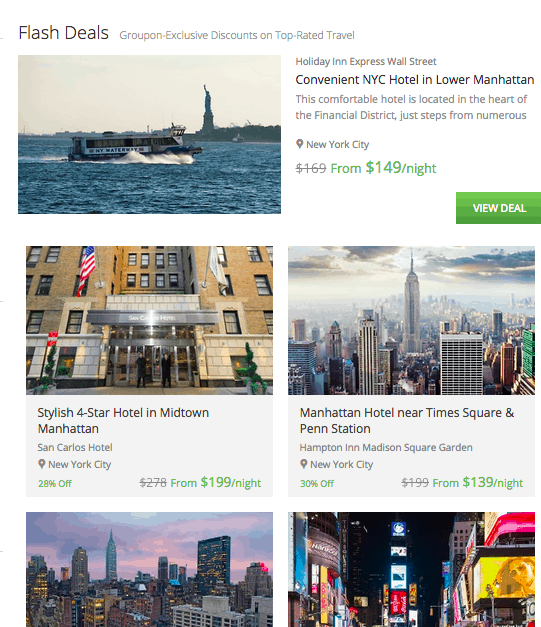### Detailed Caption:

The image depicts promotional information about various hotels, featured under the heading "Flash Deals" in bold black font. Right below this header, the text "Groupon Exclusive Discounts on Top Rated Travel" follows, with all words capitalized except "on."

The content is organized into two primary columns of text and images. In the first section, an image of a tour boat with "water something" written on its side sails through the waters around the Statue of Liberty. The accompanying text reads:

"Holiday Inn Express, Wall Street: Convenient NYC Hotel in Lower Manhattan. This comfortable hotel is located in the heart of the financial district, just steps from numerous attractions." Further details mention "New York City," indicating a previous rate of $169, now discounted to "from $149 a night" in green text, with a "view deal" option.

Below this listing, another entry describes a "Stylish, four-star hotel in Midtown Manhattan," specifically the San Carlos Hotel. Adjacent to it is another hotel description: "Manhattan Hotel near Times Square and Penn Station, Hampton Inn, Madison Square Garden."

The subsequent row features a skyline image, likely depicting New York City. Following this, there is a nighttime photo that appears to be Times Square, capturing the vibrant energy of the area.